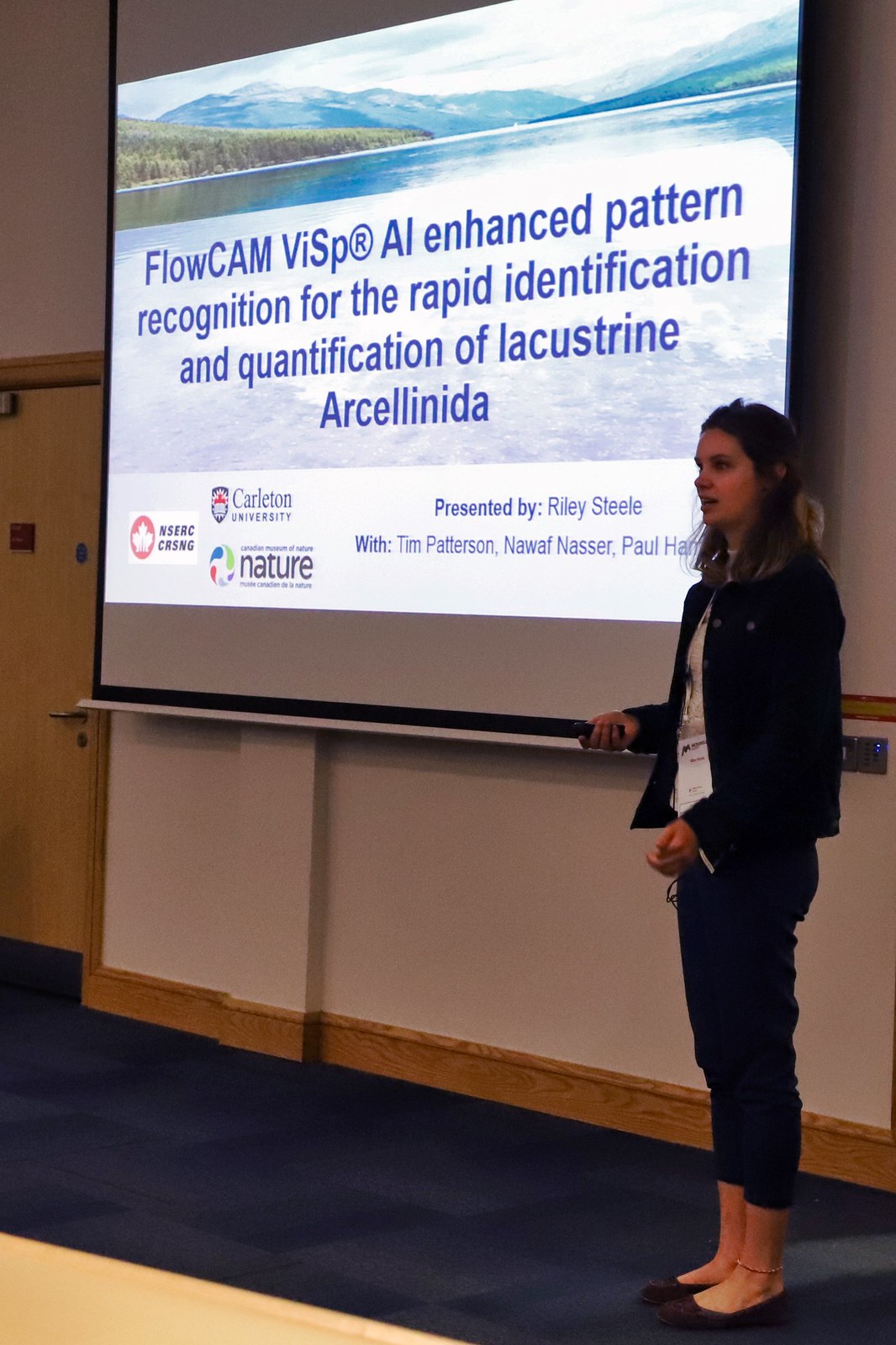In this image, we see a young Caucasian woman, presumed to be Riley Steele, giving a presentation. She stands on the right side of the frame in front of a large TV-like display or projection screen that features an image of a vast lake surrounded by mountains under a blue sky with white clouds. Some greenery is visible in the background. Riley is wearing a long-sleeve navy blue jacket over a white t-shirt, paired with black pants and black flat shoes. She holds a clicker in her hand to change the slides. The projection screen displays the title "FlowCam Vispa: Registered AI Enhanced Pattern Recognition for the Rapid Identification and Quantification of Lachustrin Arkelinida," alongside various logos including Charleston University. The presentation is credited to Riley Steele, with Tim Patterson, Nawaf Nasser, and another author whose name is partially obscured. Also, Riley is standing on a dark blue carpet.